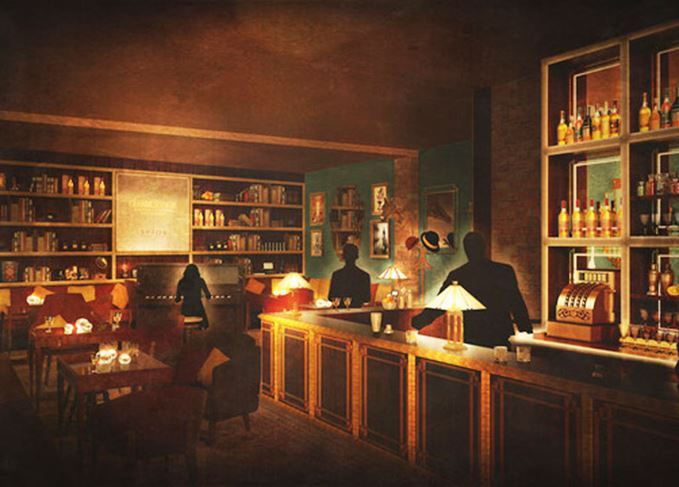This painting depicts the interior of an upscale, art deco-style bar imbued with a warm, almost supernatural glow. The bar, adorned with gold and black panels and illuminated by three elegant glass table lamps along its length, stretches along the right side of the image and features an old-style, curved metal cash register. Behind the bar, high shelves stocked with various bottles of alcohol add to the ambiance. 

The bar is populated with silhouettes: a bartender facing the viewer, a patron holding two glasses near the bar’s curve, and a pianist positioned at the far left, suggesting a lively yet enigmatic atmosphere. Comfortably padded chairs are arranged around a couple of tables, lending a sense of exclusivity to the setting. The shelves not only hold alcohol but also books, hinting at a sophisticated environment where patrons can indulge in both spirits and literature. The entire scene is bathed in muted browns, woods, and golds, exuding a cozy, inviting feel that suggests this is a high-end club or bar where art and decor speak to refinement and taste.